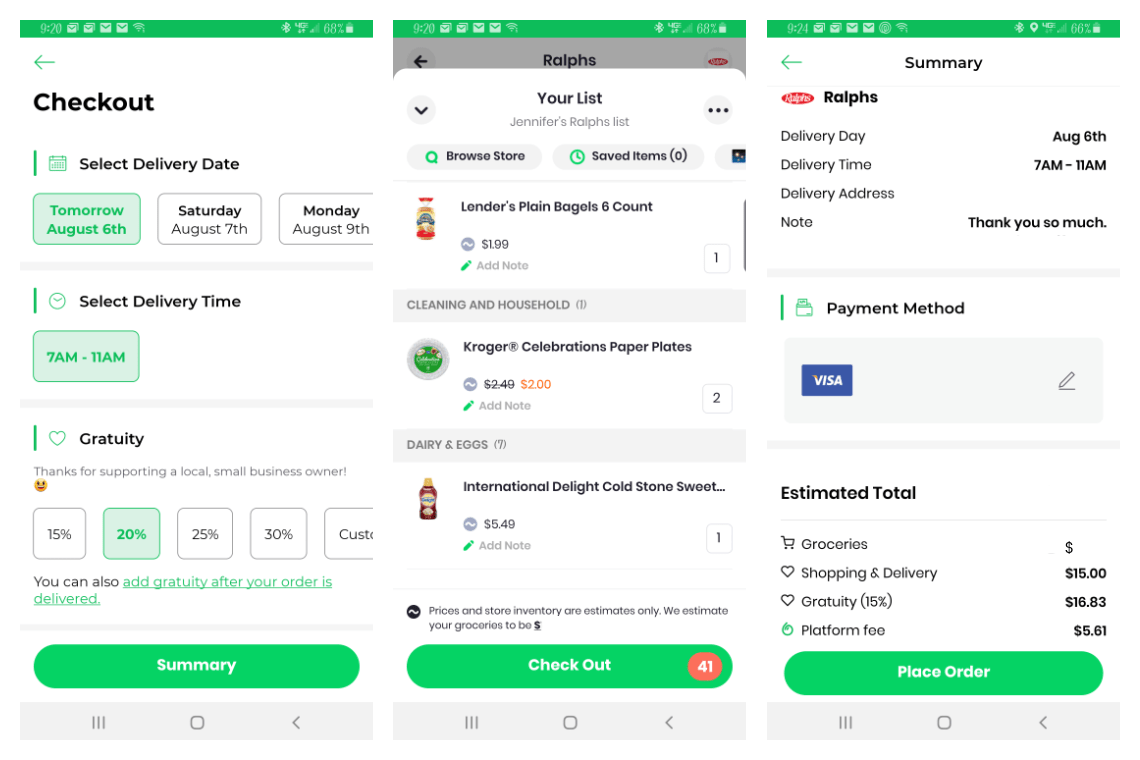In the screenshot, three smartphones are displayed side-by-side, each featuring a thin green border across the top of their screens. Along the top of each phone, there is a white timestamp on the left, followed by email icons, a battery icon displaying 60%, and a Wi-Fi/internet icon.

#### Left Phone Screen:
- **Upper Section:**
  - Large black arrow pointing left.
  - Text: "Check Out"
  - Subtext: "Select Delivery Date"
- **Tabs:**
  - First tab: Gray with green lettering.
  - Next two tabs: White with black lettering.
- **Content:**
  - Thin line
  - Text repeating: "Select Delivery Date"
  - Gray tab with green lettering followed by a thin gray bar.
  - Green heart outline with a white interior and black text labeled "Gratuity".
  - Options for tips including four predefined choices and a custom option.
  - Beneath tips: Black lettering with text "You can also" and green text "add gratuity as your order is delivered".
  - Green tab spanning across labeled "Summary" in white.

#### Center Phone Screen:
- **Heading:**
  - Text: "Your List"
  - Subheading: "Jennifer Ralphs Lists"
- **Tabs:**
  - Left tab: Gray with black text "Browse Stores".
  - Right tab: Gray with black text "Saved Items".
- **Shopping List:**
  - Item: Bagels with price
  - Item: Kroger paper plates with price
  - Category: Dairy and Eggs with other listed items including "International Delight Stone Cold Sweet Tea" and respective prices.
- **Bottom Section:**
  - Green tab labeled "Checkout" in white.
  - Red circle with "41" in white next to the green tab.

#### Right Phone Screen:
- **Screen Content:**
  - Text: "Summaries"
  - Store: "Ralphs"
- **Delivery Details:**
  - Delivery date, time, address, and note.
- **Payment Method:**
  - Visa icon indicating payment method.
- **Order Summary:**
  - Sections including estimated total groceries cost, shopping and delivery fee, gratuity, and platform fee.
- **Bottom Section:**
  - Green tab labeled "Place Order" in white.